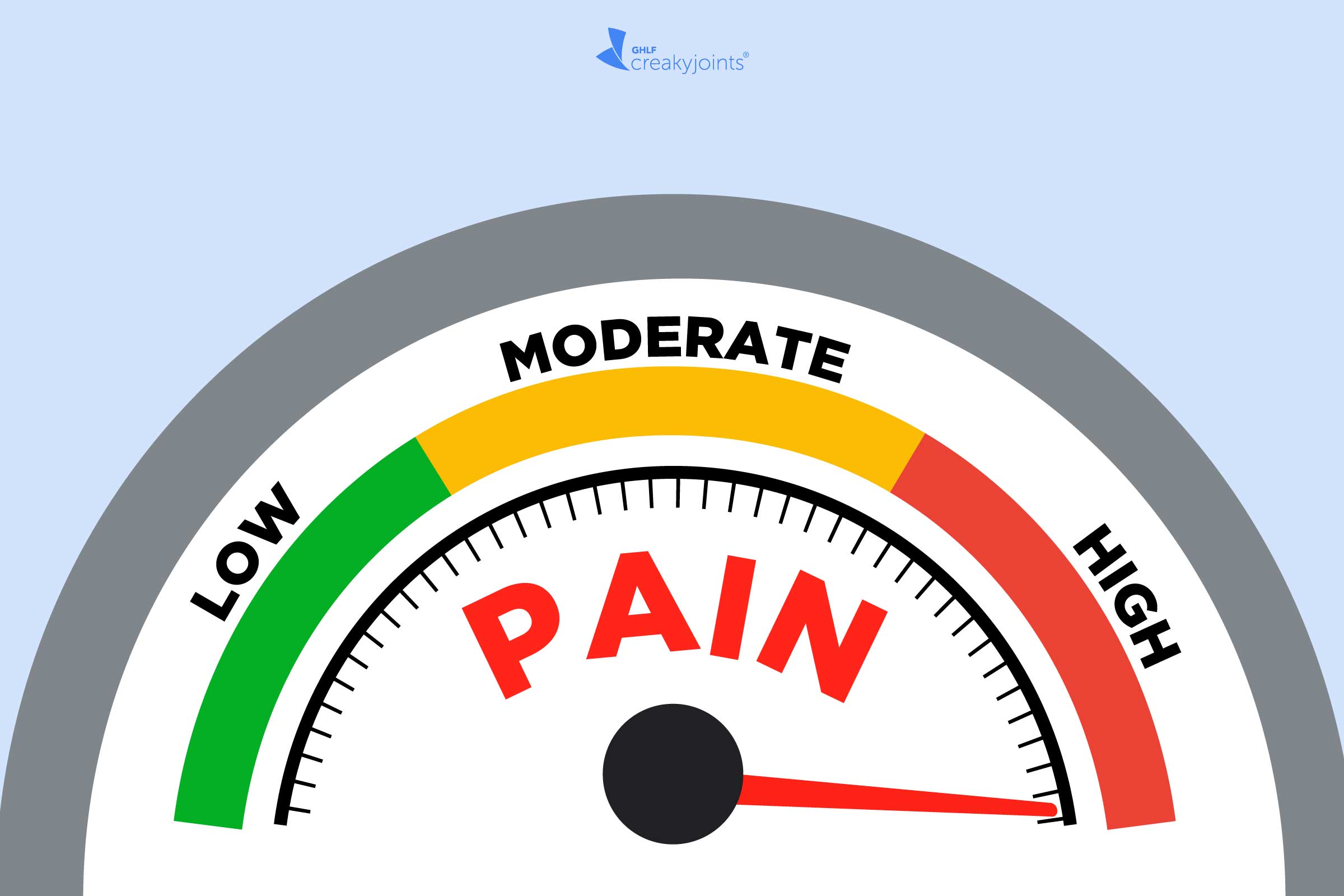This image is set against a solid light blue background that occupies the majority of the space. At the top of the image, the logo of GHLF Creaky Joints is displayed, featuring two dark blue swooshes. The central focus is a speedometer-like gauge, giving off a clip art aesthetic that suggests it was computer-generated. The gauge consists of an outer gray semicircle and an inner white semicircle, bordered by a gray ring. Dividing the gauge into three sections, the leftmost third is colored green and labeled "Low," the middle third is yellow and labeled "Moderate," and the rightmost third is red and labeled "High." In the center of the gauge, a red pointer (or needle) extends towards the segmented color bands, currently pointing to the "High" red section. The gauge also features a black circle at its center and the word "pain" written in red in the middle. Surrounding the needle are black lines resembling the numerals on a speedometer, indicating incremental levels on the gauge.